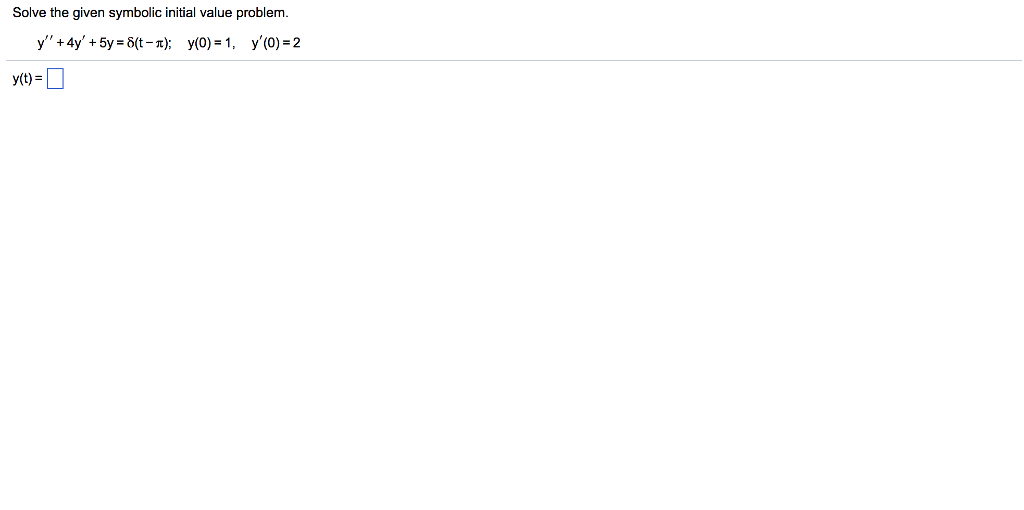The image is straightforward and primarily textual. Against a white background, the text appears in black font and reads: 

"Solve the given symbolic initial value problem:
\[ 
\frac{d^2Y}{dT^2} + \frac{dY}{dT} + 5Y = 8(T - X); \quad Y(0) = 1; \quad \frac{dY}{dT}(0) = 2 
\]

Below this, a gray line extends horizontally. Under the line, there is text that states 'Y =', followed by a blank blue-outlined box designated for the solution. 

The implied task is to solve the above differential equation, given the specified initial conditions, and to write the resulting function \( Y(T) \) into the blank box. This is the sole content of the image."